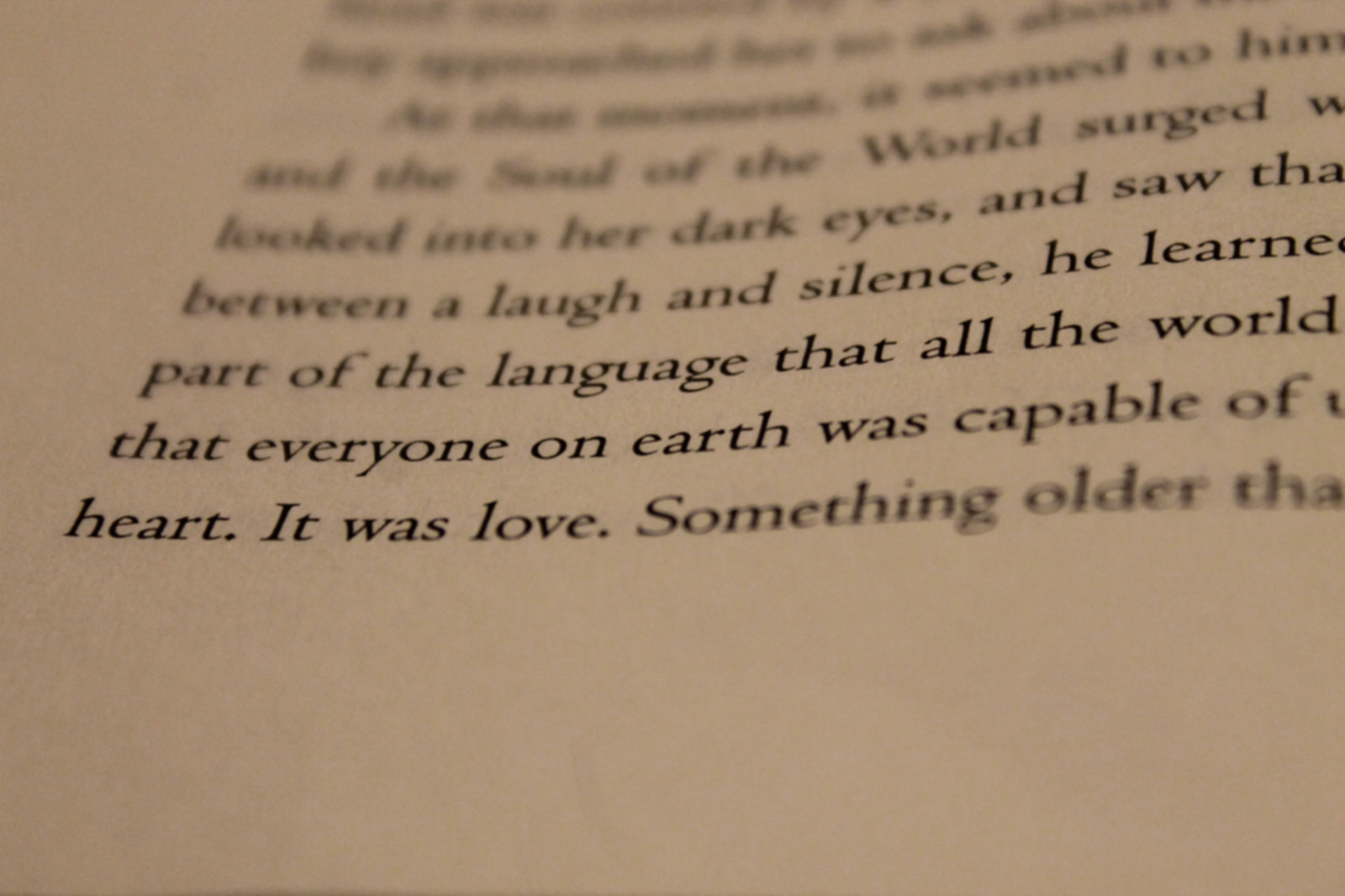This image captures a photograph of a portion of a printed page set against an off-white, light brown, or tan background, suggesting it might be tinged due to poor lighting. The background appears textured like paper, with the upper portion out of focus, indicating a close-up shot rather than a scan. The lower part of the image is blank, save for scattered, fragmented text positioned mainly in the upper right. The text includes partially legible phrases such as "soul of the world surged," "looked into her dark eyes," "between a laugh and silence, he learned," "part of the language that all the world," and "everyone on earth was capable of heart; it was love... older than." The text is fragmented, with many words cut off or blurred, making the full context difficult to discern. The visible portion suggests a narrative possibly imbued with philosophical or poetic elements.